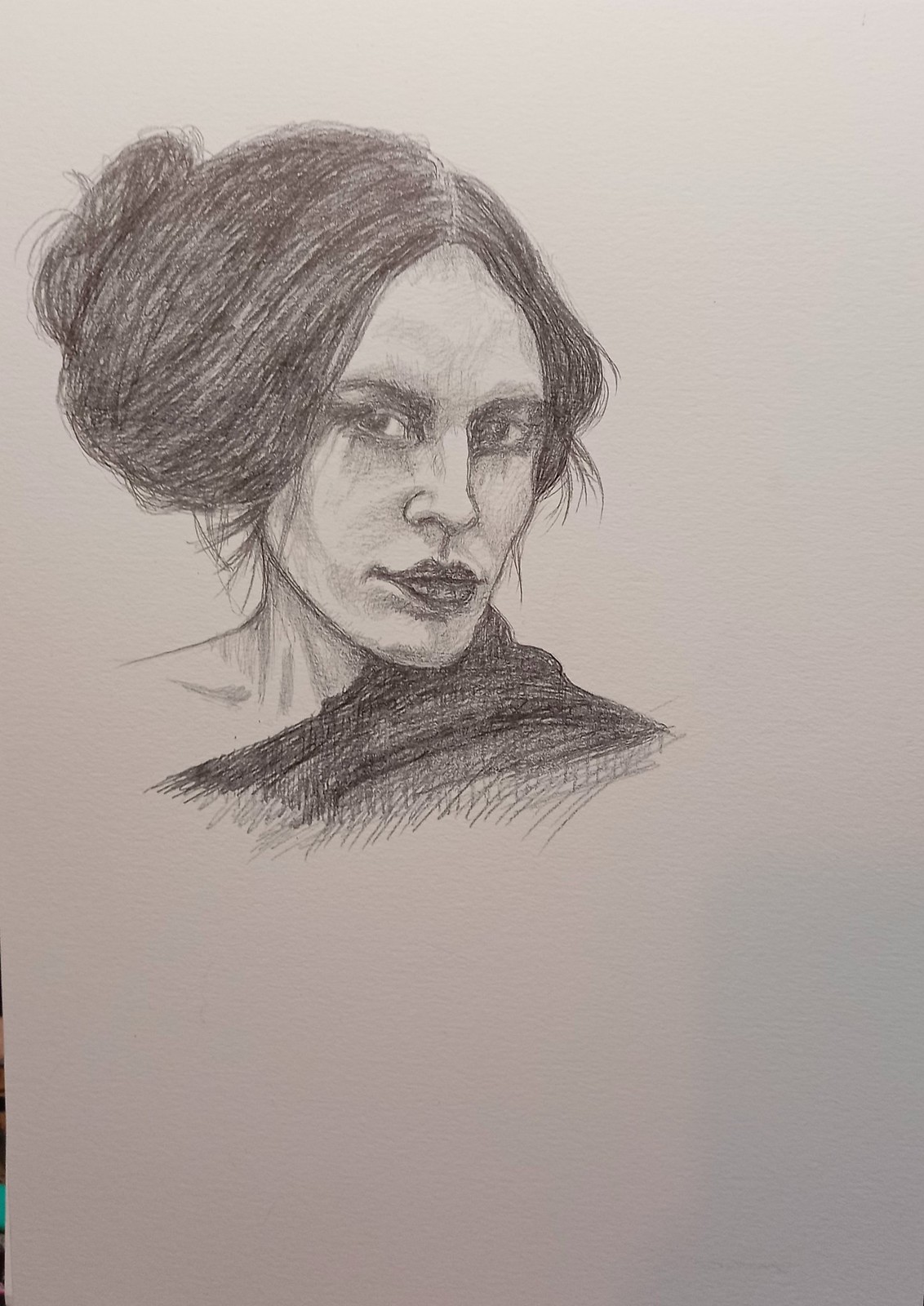This detailed pencil or ink drawing on white paper depicts an attractive, middle-aged woman with dark hair, possibly black or dark brown, that is parted in the middle and pulled back into a bun, with a few strands of hair sticking out. She has a long forehead, low, black eyebrows, and dark eyes that gaze slightly off to the side. Her full lips are shaded dark, and there is significant shading around her nose and eyes, giving her eyes a particularly dark appearance. The composition reveals just her head and neck, with a bare left shoulder while the right side is covered by what seems to be a shawl, indicated by intricately drawn lines and shading below her sharp chin. The drawing focuses on the face and the suggestion of the shoulder area, leaving the rest of her body out of the frame.